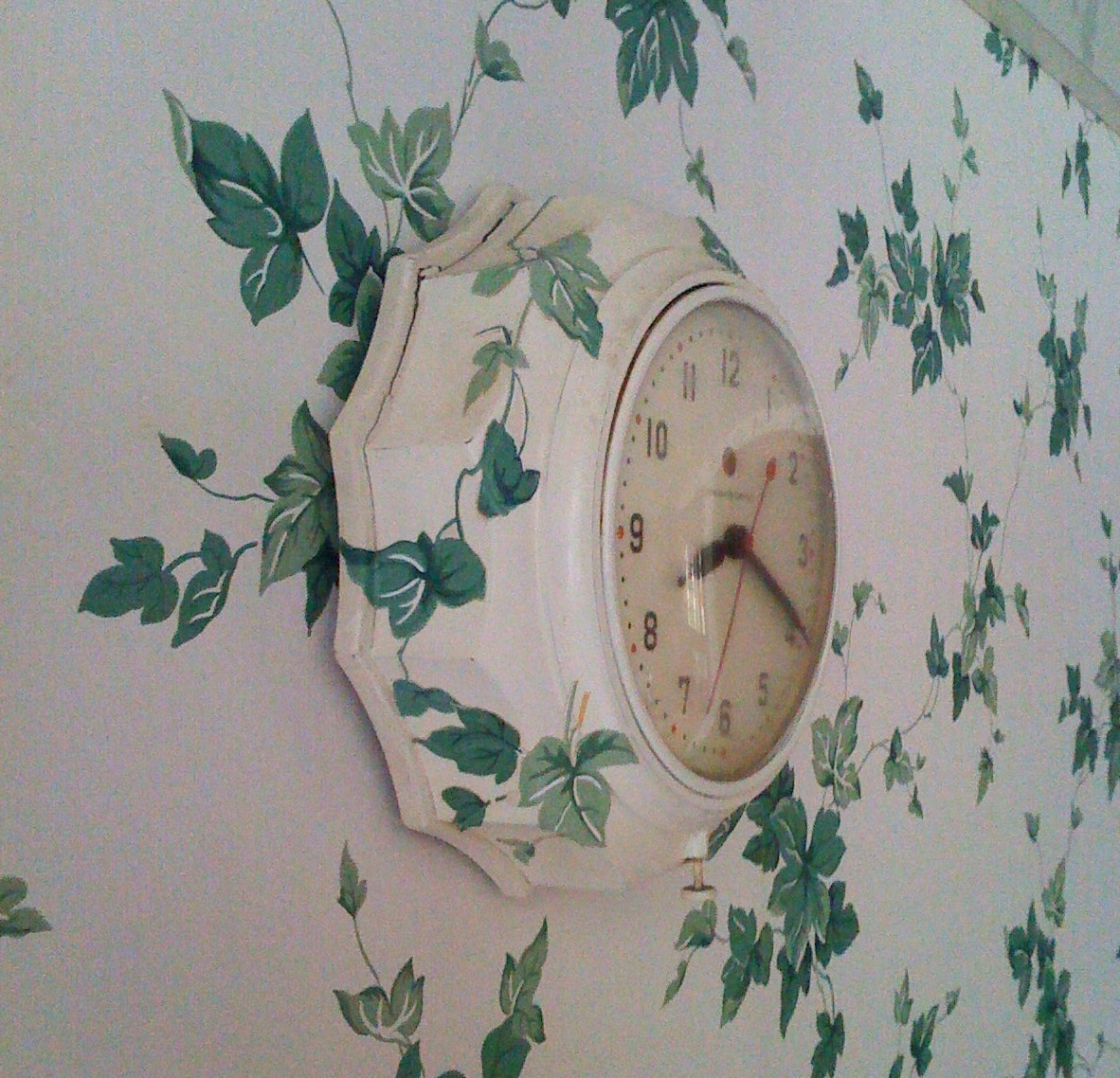This image features a circular wall clock prominently mounted on a wall. The clock has a white frame adorned with green floral designs, perfectly matching the wallpaper behind it. The wallpaper shares the same white background with green flower patterns, creating a harmonious and coordinated look. The clock face displays three hands: a short black hand indicating the hour, a long black hand indicating the minutes, and a slender red hand marking the seconds. The time shown on the clock is 8:20. The overall aesthetic is cohesive, with the clock blending seamlessly into the floral-themed decor of the room.